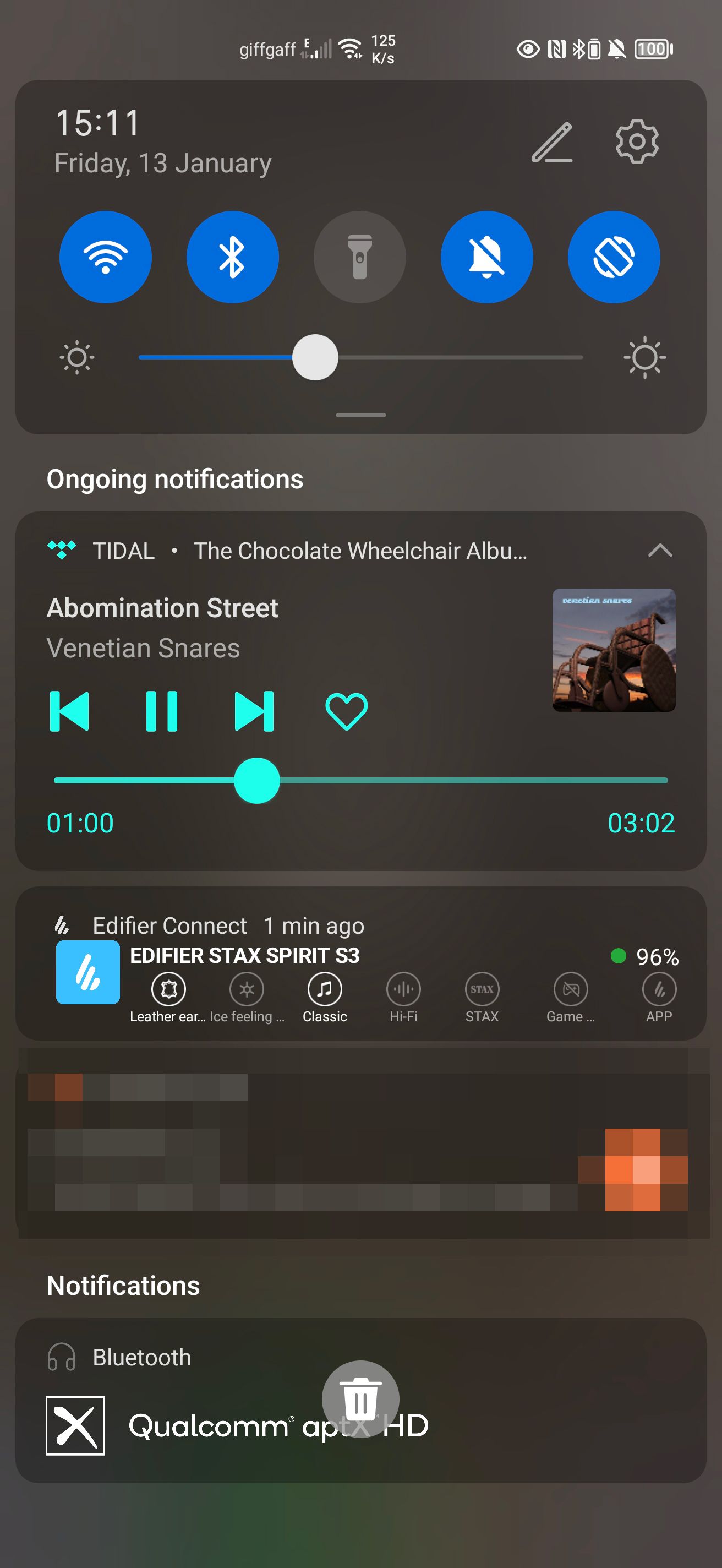This image is a detailed screenshot of a mobile phone displaying various notifications and status icons at the top. At the very top, there's a status bar with signal and Wi-Fi indicators, both at full strength. The time displayed is 1:25 with "K/S" noted next to it. Additionally, the icons for an eye, Bluetooth, a bell, and a full battery (displayed as two batteries) are visible.

Below this bar, the date and time are clearly shown as “15:11, Friday 13 January.” Two icons for editing and settings are also present in this section. 

Subsequent to the date and time, there is an ongoing notification set against a slightly grayed-out background, which transitions into a darker area showcasing an album titled "The Chocolate Wheelchair Album." 

The screenshot includes the album cover with a progress bar indicating the playback time at 1:02 out of a total of 3:02. Below the progress bar, the text reads "Edifier Connect," followed by items labeled "Edifier Stax Spirit" priced at three dollars. Details become blurred in this section.

Towards the bottom of the screenshot, there is another notification segment with a trash can icon in the center for deleting notifications.